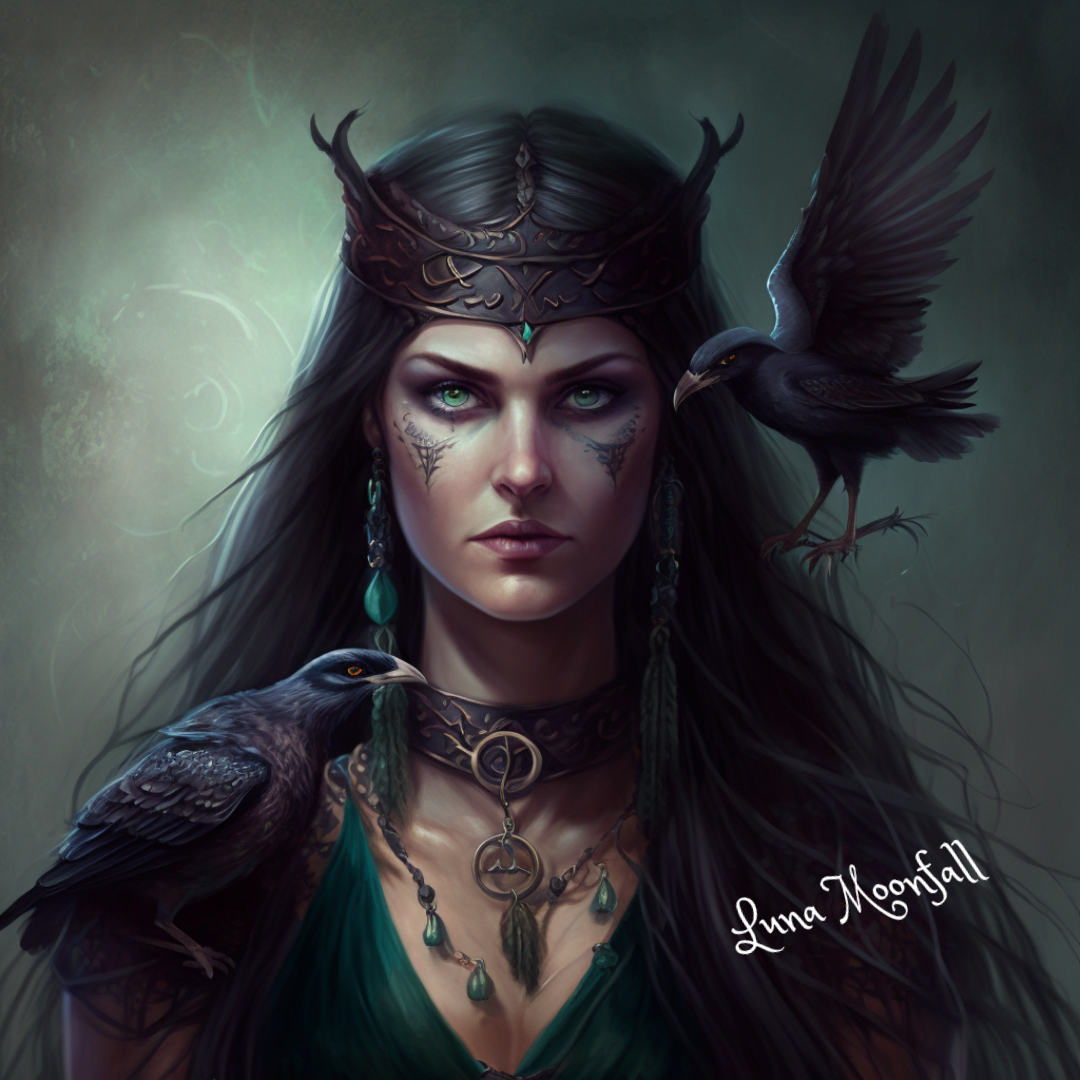This detailed artwork, reminiscent of a graphic novel or comic book illustration, showcases a stern and serious woman warrior staring directly at the viewer. The woman, with long, straight black hair, is adorned in a dark metallic tiara that resembles a crown with horn-like protrusions, and she wears elaborate jewelry, including a band around her neck with an emerald-like necklace and long earrings. Her attire features a green shirt, and her chest bears uniquely detailed skin, suggesting a fantasy or sci-fi theme to the painting. Two ravens accompany her: one hovers slightly above her left shoulder, appearing to perch on her hair, while the other is perched on her right arm. The background is an ominous blend of dark and light green hues, further enhancing the mystical atmosphere. The artist's name, Luna Moonfall, is prominently displayed in white text over the image, and her signature is located at the bottom right of the piece.